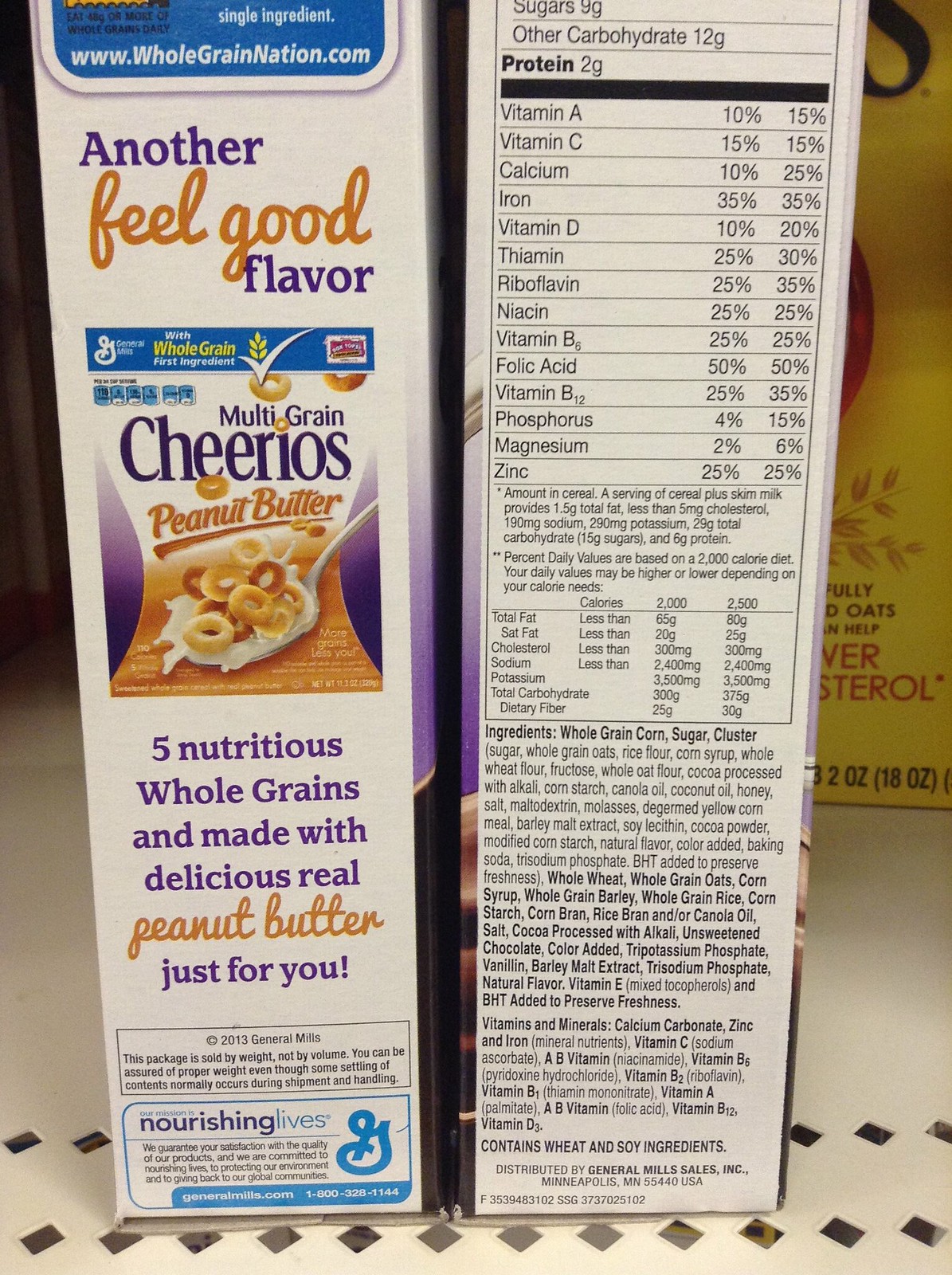This color photograph captures two cereal boxes positioned side-by-side on a white metal shelf, each showing a different side. Both boxes are of Multi-Grain Cheerios Peanut Butter flavor.

The box on the left displays promotional text starting with "www.wholegrainnation.com", followed by "Another feel-good flavor" in gold, and "Multi-Grain Cheerios Peanut Butter" in purple. It boasts "Five nutritious whole grains made with delicious real peanut butter just for you." General Mills information, including copyright 2013, weight assurance, mission statement, satisfaction guarantee, and contact details (Generalmills.com, 1-800-328-1144) are detailed below. 

The box on the right, partially cut off at the top, highlights the nutritional information, listing sugars as 9 grams, other carbohydrates 12 grams, and protein 2 grams. It details the vitamins and minerals included: vitamin A 10%, vitamin C 15%, calcium 10%, iron 35%, vitamin D 10%, thiamine 25%, riboflavin 25%, niacin 25%, vitamin B6 25%, folic acid 50%, vitamin B12 25%, phosphorus 4%, magnesium 2%, and zinc 25%. Below this nutritional information, the ingredients list is visible, noting it contains wheat and soy, and is distributed by General Mills Sales Incorporated, Minneapolis, MN 55440 USA.